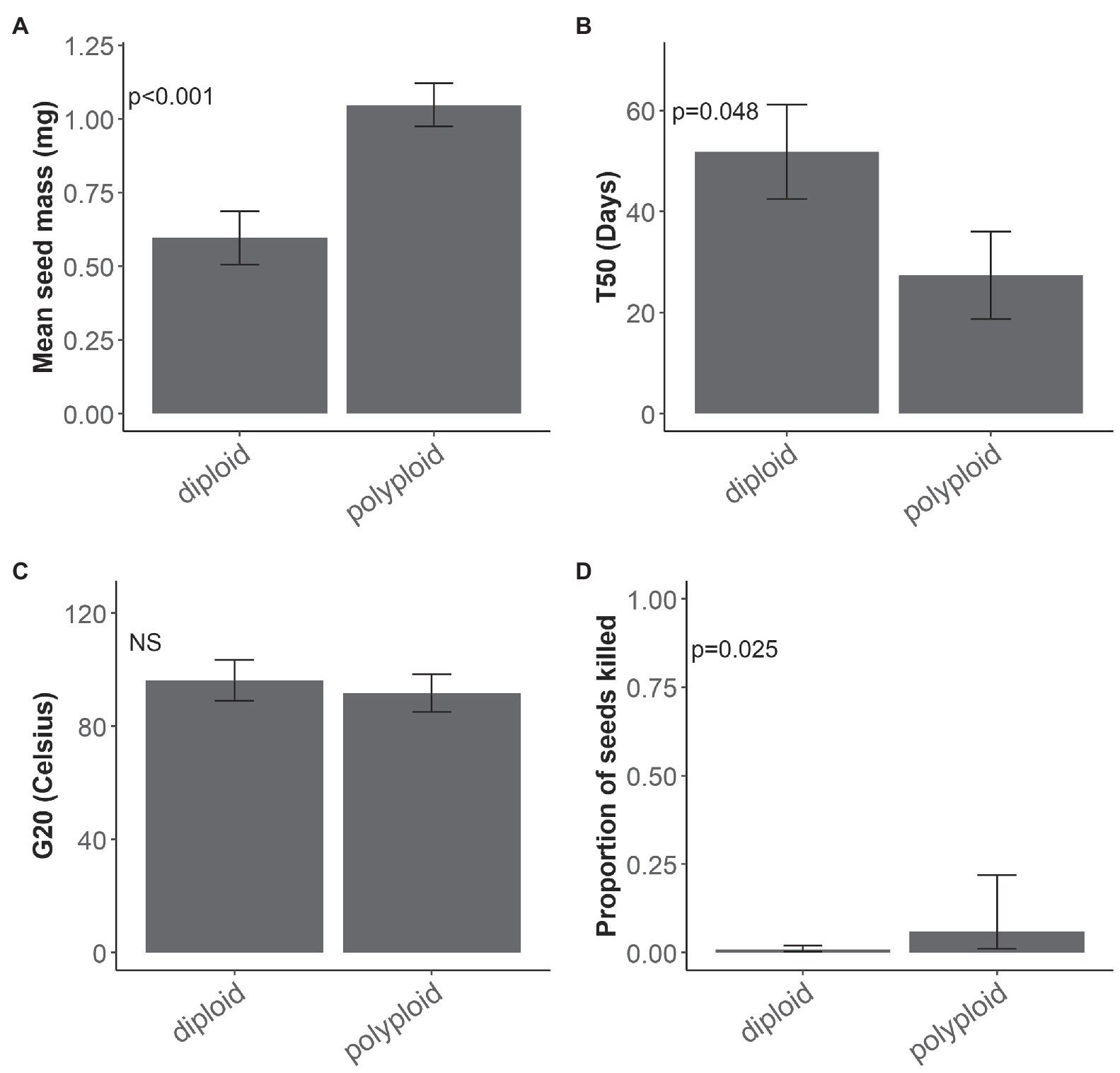The image features four detailed bar graphs arranged in a 2x2 grid, labeled A, B, C, and D. Each graph is presented in grayscale, with two thick bars indicating data points for diploid and polyploid categories. 

- **Graph A**, located in the upper left, is titled "Mean Seed Mass (MG)." It measures from 0 to 1.25 and displays a short thick bar for diploid and a tall thick bar for polyploid.
- **Graph B**, positioned in the upper right, is labeled "T50 Days" and scales from 0 to 60. This graph shows a tall thick bar for diploid and a much shorter thick bar for polyploid.
- **Graph C**, found at the bottom left, is titled "G20 (°C)" with a range from 0 to 120. It depicts two fairly tall thick bars of nearly equal height for both diploid and polyploid.
- **Graph D**, in the bottom right, is labeled "Proportion of Seeds Killed," scaling from 0 to 1.25. It features an almost negligible bar for diploid and a very short bar for polyploid.

Each graph includes precise numerical scales and labels, providing a clear visual comparison of the characteristics measured between diploid and polyploid samples.